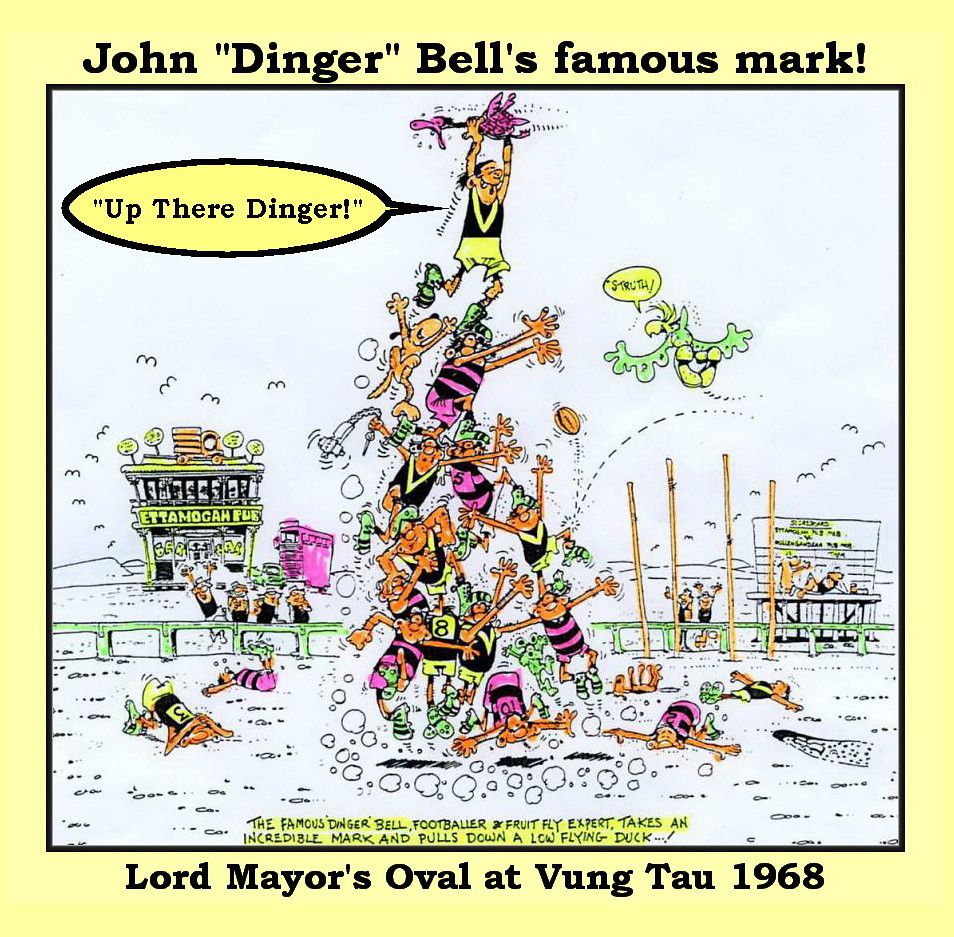The image appears to be a hand-drawn, artistically created poster, potentially derived from a comic strip, showcasing an event. It is bordered by a light yellow or tannish frame that reads, "John 'Dinger' Bell's Famous Mark!" at the top, and "Lord Mayor's Oval at Vung Tau, 1968" at the bottom. Dominating the center of the image is a chaotic yet humorous scene of people stacked in a human pyramid, with some individuals laying awkwardly on the ground, suggesting failed attempts or exhaustion. The person at the top of the pyramid has a thought bubble saying, "Up There, Dinger." Scattered among the people are whimsical elements such as a purple bird, a bird with a text bubble saying "Is truth!" and an orange Snoopy. Several individuals wear shirts with numbers, including a pink and black striped number 10, contributing to the playful vibe. In the background, a store can be seen along with distant buildings, adding depth to the setting. The color palette includes yellow, black, white, pink, purple, orange, green, and gray, enhancing the lively and comic atmosphere of the scene.